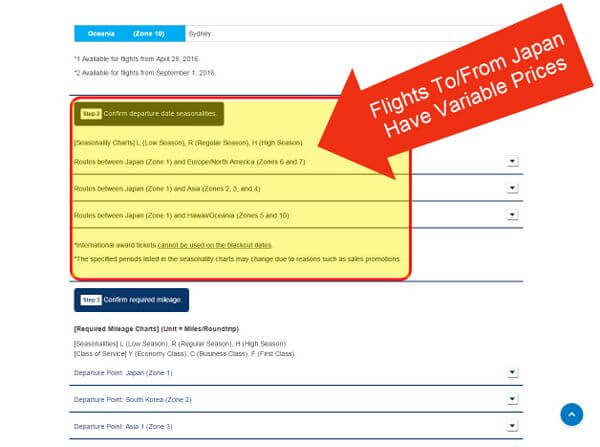Category: Websites

Caption: This image depicts a small, low-resolution chart related to travel routes and required mileage points. Due to its size, the text is difficult to read and cannot be expanded without significant blurring. The top of the chart features a blue header, which likely reads "Oceana Zone." Below the header, various sections outline the requirements for confirming departure dates along with the different seasons categorized as Low Season, Regular Season, and High Season. Specific route information is provided, detailing travel between Japan (Zone 1) and other regions: Europe and North America (Zones 6 and 7), Asia (Zones 2, 3, and 4), and Hawaii (Zones 5 and 6). Additionally, the chart appears to include information about the required mileage, perhaps under a section labeled "Required Mileage Charts," with units measured in miles for round trips.